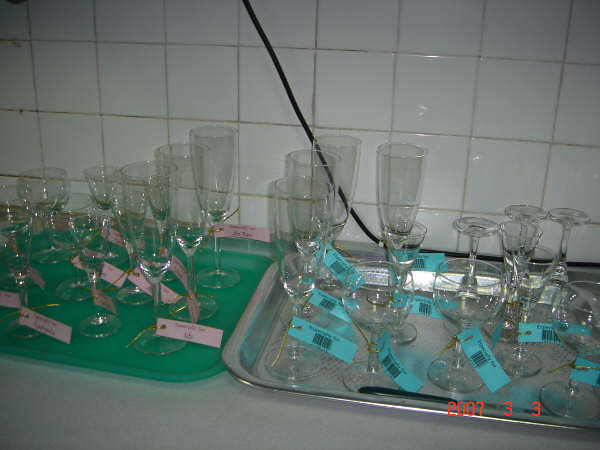This detailed photograph, taken indoors, captures a meticulously arranged scene on a light gray surface. The back wall, featuring a grid of cream-grouted, white 4x4 inch tiles, consumes approximately half of the image. Two trays dominate the lower half: a green tray on the left and a stainless steel one on the right, each laden with an assortment of wine glasses, champagne flutes, cordial glasses, and water glasses. Adorning the glasses on the green tray are pink tags fastened with gold metallic twisty ties, while turquoise blue tags, some displaying black barcodes, are affixed to the glasses on the stainless steel tray. At the bottom right corner, the date "2007 3 3" is displayed in red text, reminiscent of a timestamp from a digital camera.